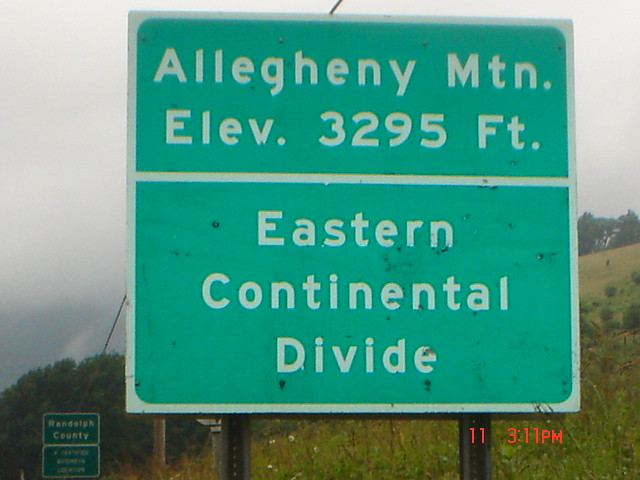This photo captures a large green and white highway sign, which is square and mounted on two sturdy white metal posts. The sign prominently reads: "Allegheny Mountain Elevation 3295 feet Eastern Continental Divide." A date stamp at the bottom right corner of the image in red text indicates "11" followed by a time stamp of "3:11 p.m." The background reveals a grassy slope that begins mid-way on the right side and extends towards the bottom left. The grass, which is green to light green, suggests a hill or incline. An overcast sky looms above, heavy with gray clouds that give the impression of imminent rain. In the lower left of the image, there is an additional street sign at a distance, partially out of focus and difficult to read, though it states "Randolph County." The photo is characterized by a graininess and haziness, contributing to the dim illumination typical of an overcast day. The left and right corners of the scene contain clusters of trees, reinforcing the natural, rural setting.